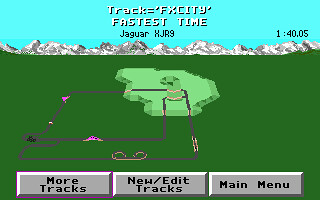The screenshot features a retro-style, 2D pixelated video game, reminiscent of classic arcade racing titles. The image, taken from a small display with no visible background, highlights the game's interface and elements in a detailed manner. At the top center in white text, it displays "Tracks, FX, City, Fastest Time." To the left, in black text, it reads "Jaguar XJR9," while the far right shows a fastest time of "1 minute 40.05."

At the bottom of the image, three grey rectangular buttons with black text are visible: "More Tracks," "New/Edit Tracks," and "Main Menu," from left to right. The "More Tracks" button is distinguished by a blue border, indicating it is currently selected. The game scene itself showcases a 2D race track set in an isolated green field. In the background, snow-capped mountains rise against a blue sky, where the text "Tracks, FX, City," and the fastest time are superimposed. Pixelated cars populate the race track, adding to the nostalgic, arcade feel of the image.